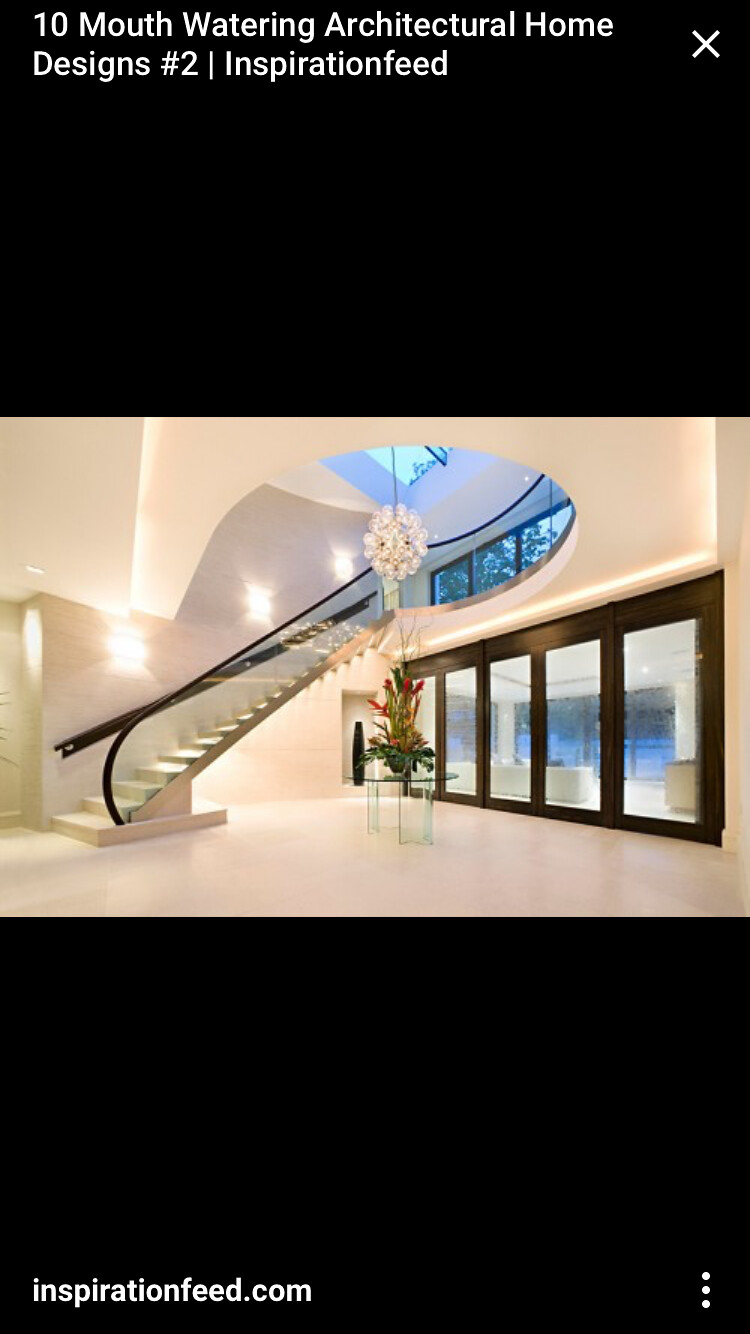This image appears to be an advertisement targeting individuals interested in home design, real estate, or architecture. Prominently displayed at the top right in white letters is the phrase "10 mouth-watering architectural home designs, number two, Inspiration Feed," hinting at a series of inspiring architectural features. The top and bottom thirds of the image have a black background, with the website "inspirationfeed.com" inscribed at the bottom. 

The central focus of the image showcases the foyer of a contemporary, sleek home characterized by its open and bright atmosphere. The room features pristine white walls and white granite flooring. A striking white floating staircase ascends to the second floor, adorned with a medium brown banister railing, creating a harmonious blend of modern and traditional elements. The staircase is accentuated by skylights that flood the space with natural light.

Beneath the staircase, a five-paneled wall composed of glass doors framed in dark brown offers a glimpse into another section of the home. Centrally located in the foyer, a chic glass table supports a large floral arrangement with red blossoms, adding a vibrant touch of nature. Overhead, a glamorous chandelier composed of spherical glass balls enhances the room's elegance. The image is devoid of any people, emphasizing the architectural and design features, and includes a distinctive trio of vertical white dots in the bottom right corner. The main colors presented are black, white, and brown.